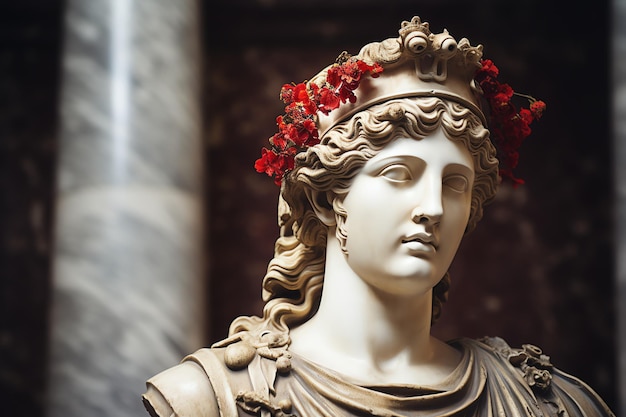This landscape-oriented color photograph features a finely carved statue of a Greek goddess situated on the right side of the image. Captured from chest upwards, the statue boasts realistic details despite its single-tone pale white hue, characteristic of marble or granite. The goddess wears a slightly ruffled and layered round-neck garment, tinged subtly in bronze or beige. Her wavy, long hair cascades down her neck and lightly rests on her right shoulder. Atop her head, a crown with dried red flowers adorns her above the hairline. Her eyes, devoid of irises, gaze slightly off to the left. Behind her right shoulder, a large, round marble column with distinctive grey and white patches stands out in soft focus, while the backdrop on her right remains enveloped in dark grey and black tones, adding depth to the composition. The impressive intricacies of her nose and mouth further exemplify the craftsmanship, making this statue a striking and detailed representation of classical art.